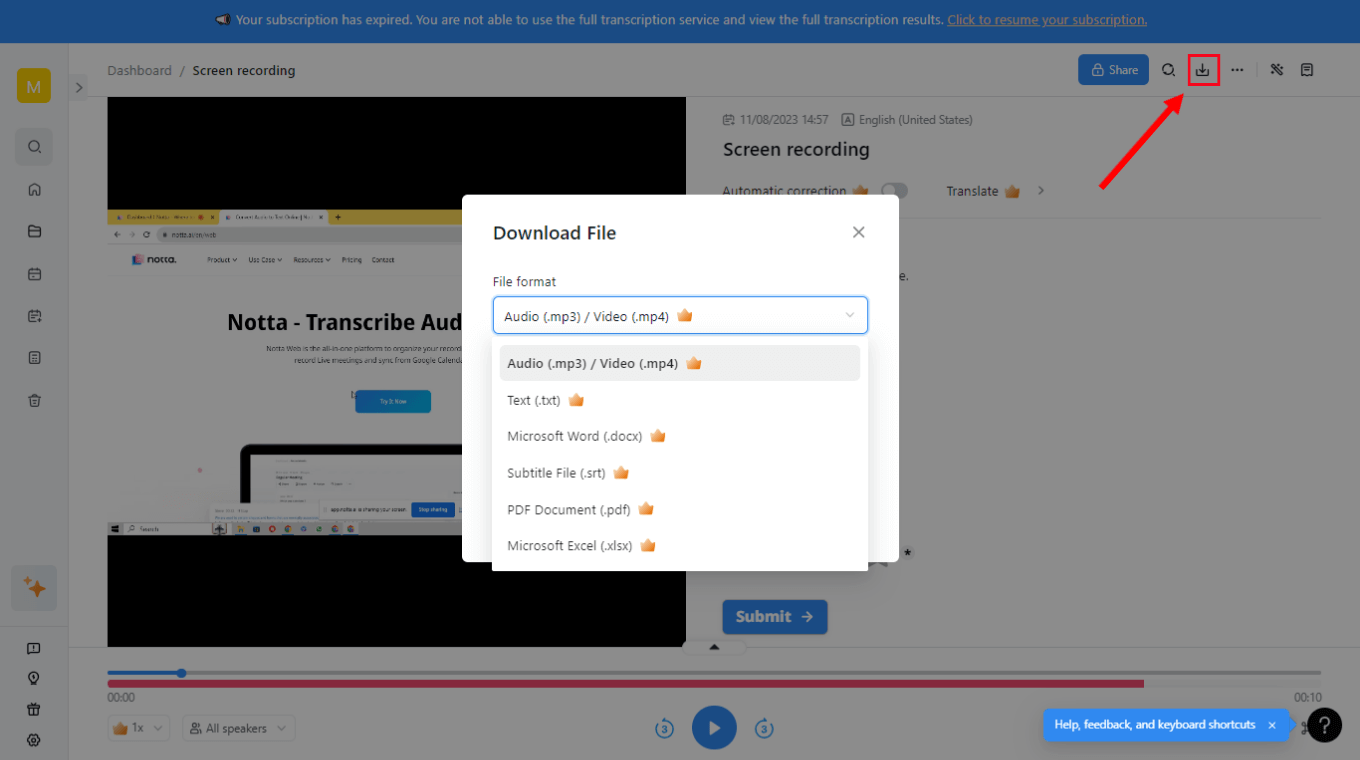Screenshot depicting a program interface for downloading a file. At the top, a prominent blue rectangle spans the entire width of the screen, notifying the user that their subscription has expired and they are unable to use the full transcription service or view comprehensive transcription results. The message within the blue rectangle is written in gray text, prompting users to click there to renew their subscription.

Below this notification, the interface is divided into several sections. On the left side, a navigation menu includes options like "Dashboard" and "Screen Recording." The main content area displays a large black rectangle, suggesting a video or screen recording. This section is labeled "Audio Format: MP3/Video" and includes a dropdown arrow revealing various file format options such as audio file, text file, Microsoft Word file, subtitle, PDF, and Excel.

A timestamp indicates a screen recording was made on November 8, 2023, at 14:57 (4:57 PM). A red square with an arrow highlights a download button, suggesting the user is in the process of downloading the stated content. The background appears dimmer compared to the bright white pop-up for file format selection, emphasizing the active selection area.